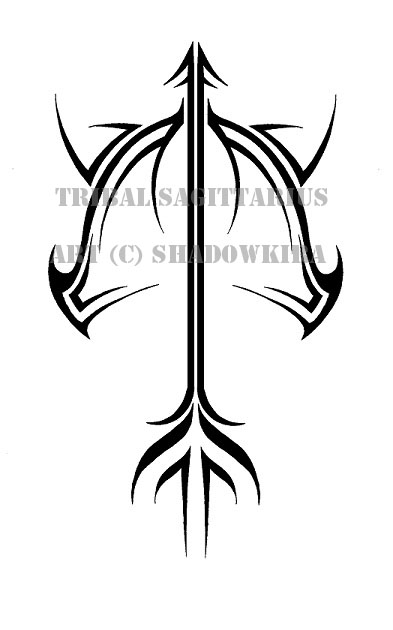This image showcases a striking example of tribal tattoo art, presented in black on a white background. At the center of the design, an arrow-like figure points upwards, resembling a loaded bow, oriented from south to north, while the bow stretches from west to east. The design is characterized by its simplicity and minimal use of lines, with each curve and edge ending in spiky points, giving it a sharp, dynamic feel. The arrow is horizontally split into two sections, and decorative elements such as feathers adorn its base. These features collectively form a design that also evokes imagery of a helmet, particularly one that might resemble a Viking helmet with a rounded top and a broad base. Overlaying this bold tribal design is a gray watermark that reads, "Tribal Sagittarius Art (C) Shadow Killa," indicating the artwork's title and copyright information. The tattoo-like composition underlines the artistic intent behind the creation, making it both a distinctive and classic piece of tribal art.